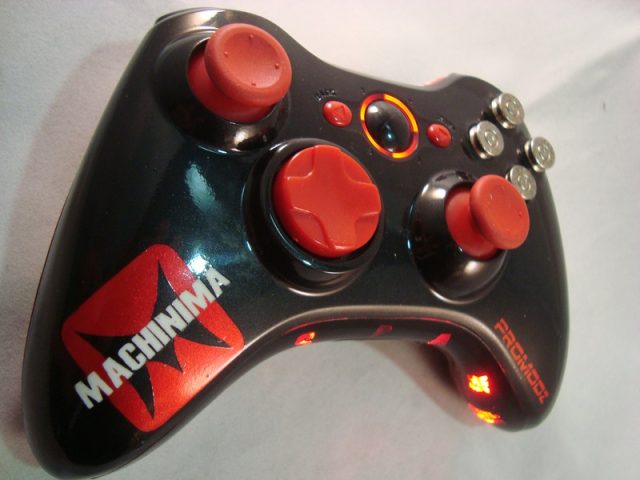This image showcases a customized vintage Xbox controller, predominantly black with red accents. The left-hand grip prominently features a red square with a stylized black "M" and the word "Machinima" in white lettering, paying homage to the well-known multi-channel network. On the right-hand grip, the phrase "Pro Mods" is showcased in red and black lettering, suggesting the controller's modified nature. The analog sticks, D-pad, and the various buttons including the start and select, are all vividly red, contrasting with the sleek black body. The buttons A, B, X, and Y have been replaced by flat, metallic silver buttons, void of any symbols. Notably, the large central button is encircled with a red and golden border, and additional red lights adorn the bottom, adding a unique illuminated touch to the design. Despite some signs of wear, the controller's intricate and bold modifications give it a distinctive vintage appeal.